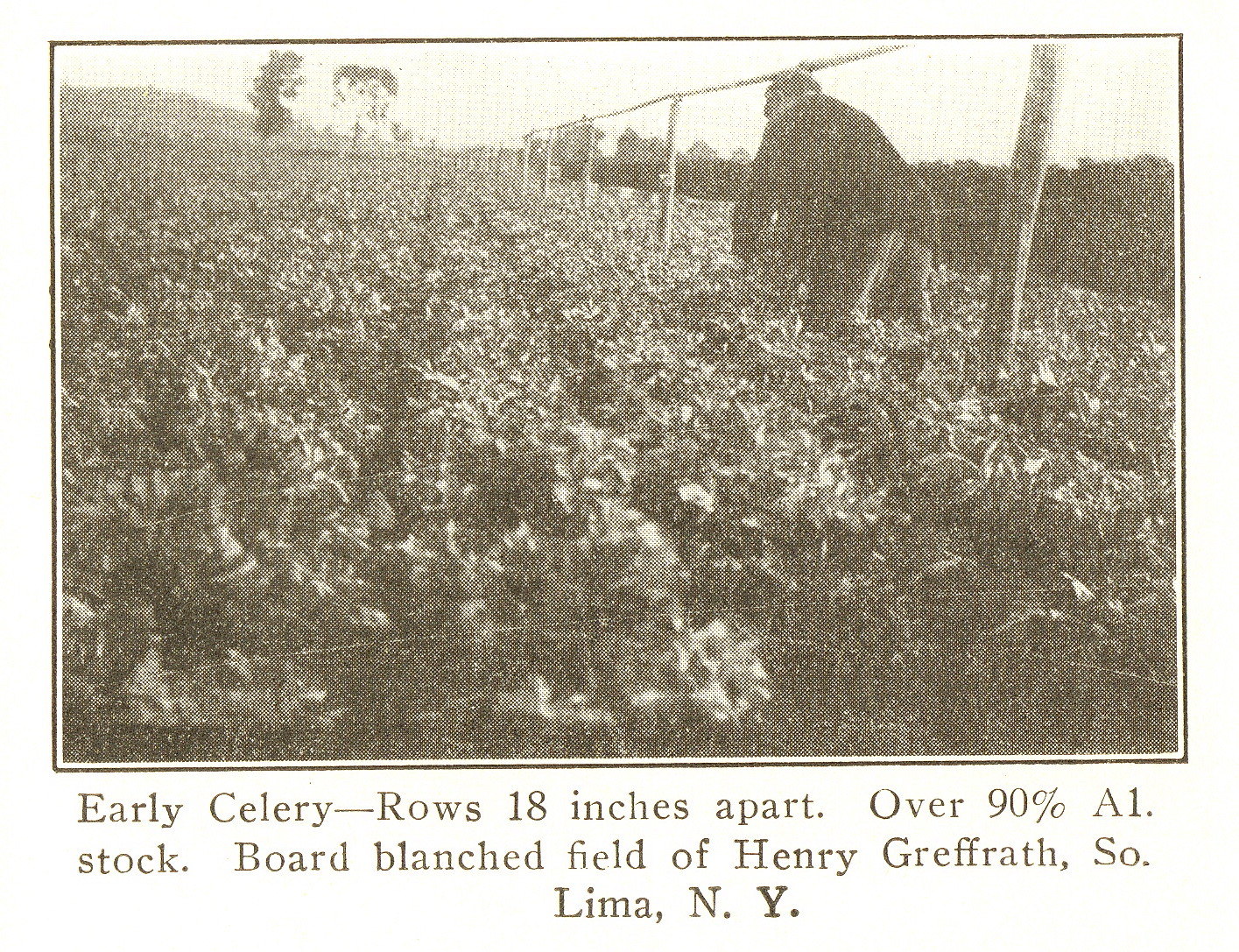This black-and-white newspaper clipping features a very old, faded photograph with a thin black border. It depicts a person, possibly a farmer, hunched over in a field of knee-high plants, likely celery, as indicated by the caption. The rows of plants are evenly spaced, 18 inches apart, extending into the background where a row of trees marks the horizon. The farmer is positioned towards the right side of the image, near a wooden fence made of wire and wooden posts. The scene captures the essence of early agricultural practices. Below the photograph, the caption in black letters reads: "Early celery, rows 18 inches apart, over 90% A1 stock, Bord Blanched Field of Henry Greffrath, South Lima, New York."